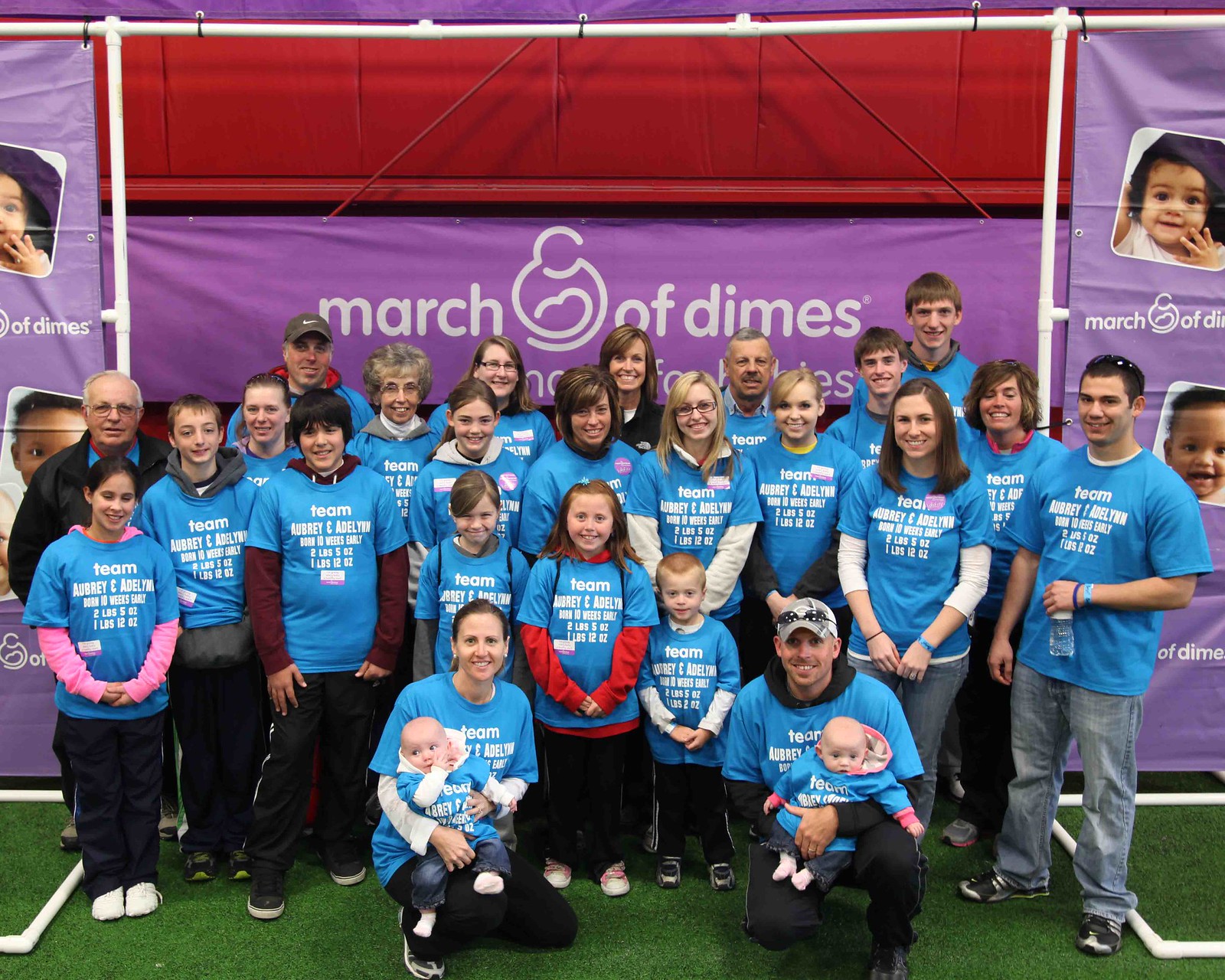The photograph captures a large group of over 20 people attending a March of Dimes event. The backdrop features a white frame holding up tall purple banners with white lettering that reads "March of Dimes," along with small square pictures of babies on either side. The group, consisting of both older adults and young children, is arranged in approximately three rows on green turf or carpet. Most of them are dressed in matching short-sleeved turquoise blue t-shirts with white text that reads "Team Audrey and Adeline," though some individuals have layered long-sleeve shirts underneath, including bright colors like hot pink and red. In the front row, a man and a woman each cradle a baby, flanked by three smiling kids. The entire group faces the camera with joyful expressions, conveying a sense of happiness and community spirit at the event.